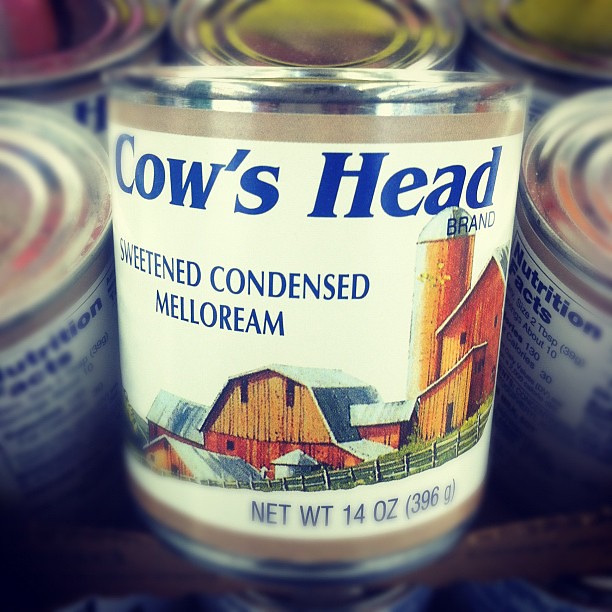A close-up photograph captures a can of "Cow's Head" sweetened condensed melloreme. The can, short and stubby, features a quaint illustration of a picturesque farm complete with a barn, silo, and additional structures. The net weight of the product is detailed at the bottom of the can, listing it as 14 ounces or 396 grams. The edges of the can blur softly into the background, revealing it as part of a group of indistinguishable, identical cans. Despite the blur, neighboring cans on either side hint at a nutrition label on the back, specifying that a serving size is two tablespoons with approximately 10 servings per can.